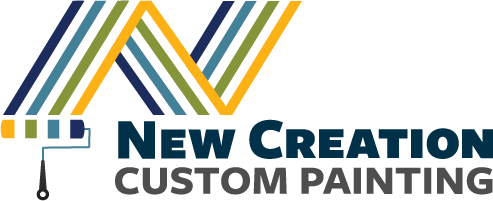The image features a company logo set against an all-white backdrop. Dominating the image are the bold, navy blue words "New Creation," with the phrase "CUSTOM PAINTING" appearing in a smaller, gray, all-caps font beneath it. The logo is complemented by a paint roller illustration in the bottom left corner, from which a series of colorful stripes flow horizontally. These stripes transition from yellow to orange, then green, followed by light blue, and culminating in a dark blue hue. These colors form the letter 'N' in a zigzag pattern across the logo, suggesting the paint roller is actively painting the 'N'. The detailed design creatively merges text and imagery to emphasize the company's focus on custom painting services.